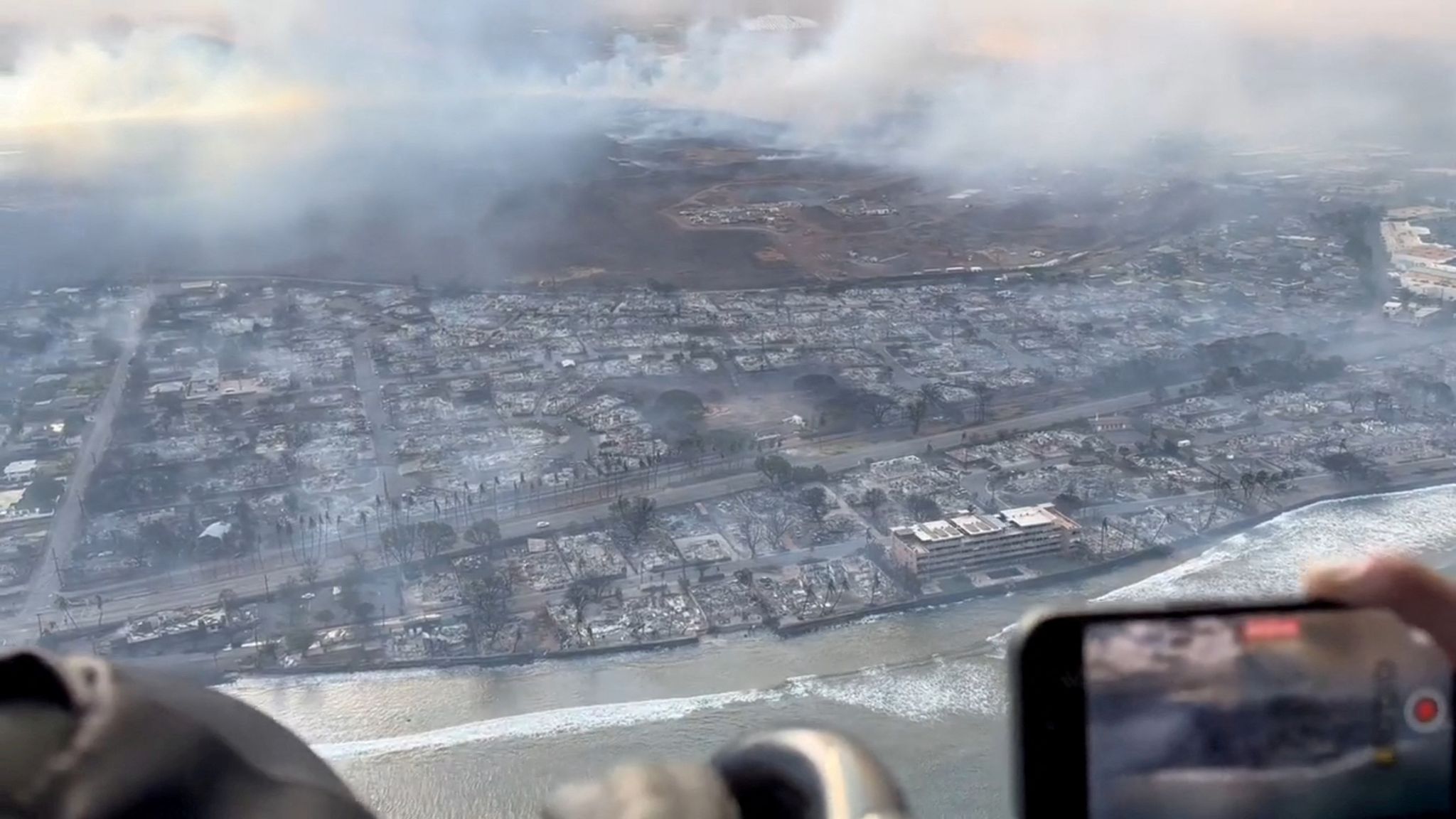This aerial photograph captures a town partially obscured by clouds, taken from within the clouds, likely from an airplane. The image reveals a densely packed cityscape with numerous buildings and roads beneath, presenting a stark contrast between areas of apparent destruction and untouched sections. The lower part of the image, particularly to the bottom right, shows a person holding a smartphone, which displays part of the town visible in the main photo, suggesting the scene is being videoed. The bottom left reveals an unknown gray object, possibly a part of the photographer's body. A beachfront borders the city with waves rolling towards the damaged structures. The scene suggests the aftermath of a wildfire, with burned palm trees and other vegetation, and a multi-story waterfront building showing visible damage. To the upper right, some clean, untouched white buildings stand out amidst the pervasive smoke and destruction, likely illustrating the 2023 wildfires in Hawaii.